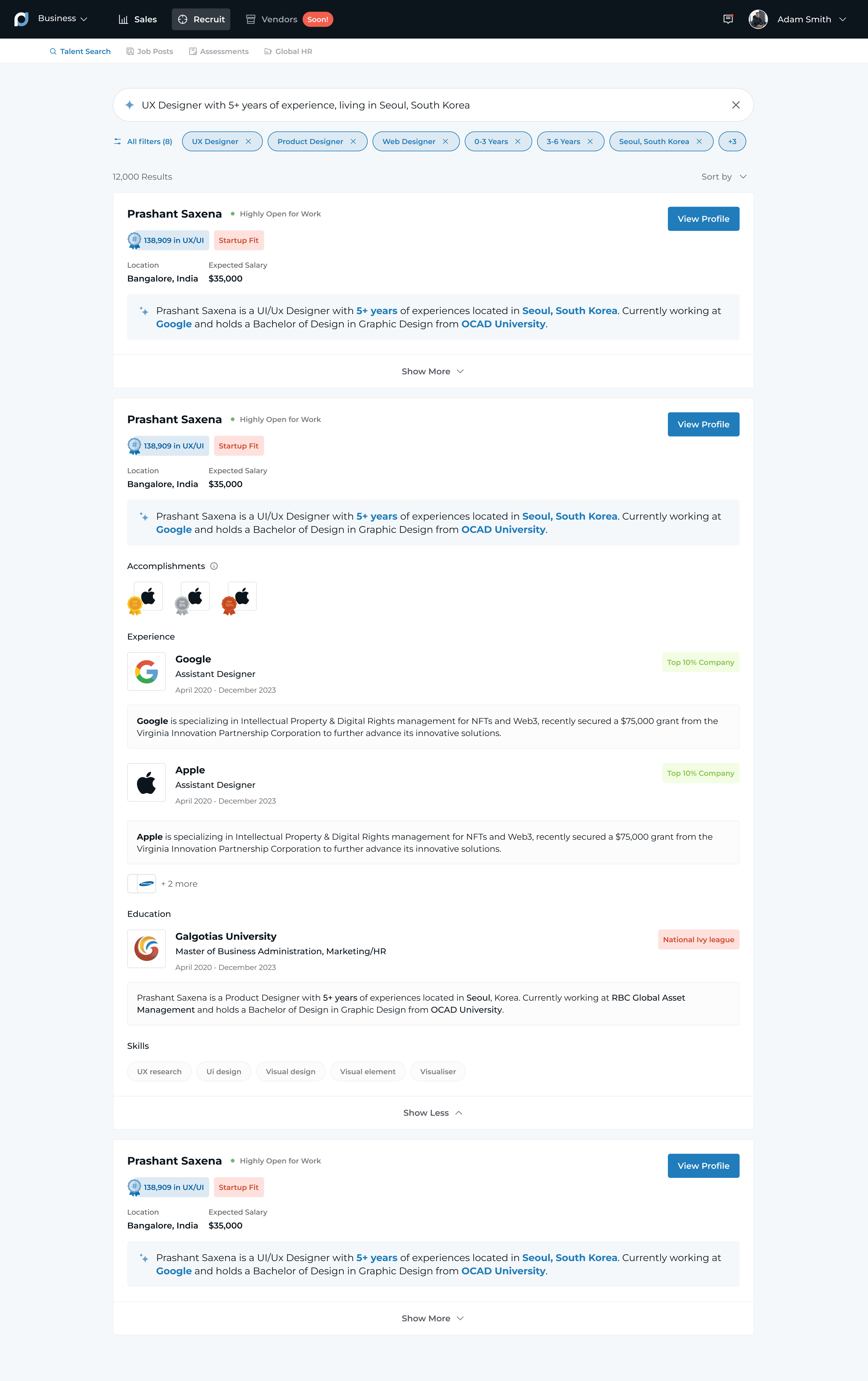The image depicts a desktop website that has been formatted for tablet view, making the text extremely small and difficult to read. The compressed nature of the text renders it nearly illegible, even when zoomed in. At the top of the page, a black bar features a symbol of a circular white and blue arrow, resembling a loading icon. Below this bar, there are three buttons, with the middle one currently selected. In the top right corner, a profile picture of a person sitting with their arms crossed is visible, alongside a legible username. The website appears to be related to a Google service, possibly showcasing account information or settings. The presence of logos for Google, Apple, and a university further supports this identification. The overall background of the page is white, contributing to the difficulty in reading the text.